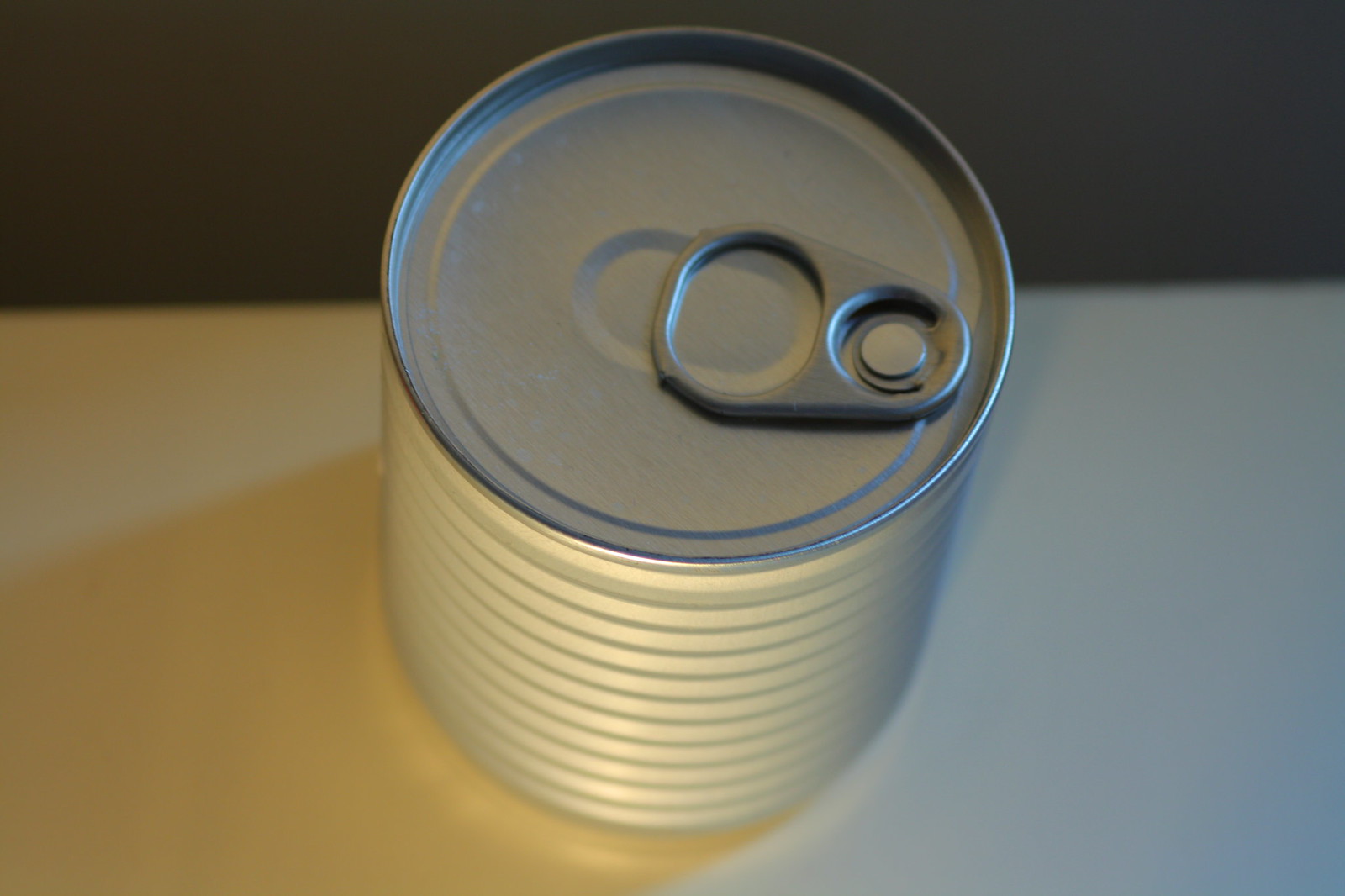This is a high-angle, real-life photograph of a closed, unlabeled metallic can. The can's top, which gleams with silver tones, features a pull-tab for opening. The cylindrical body of the can showcases characteristic ridged lines encircling it, giving structure to the product. Resting on a light off-white surface, the can casts a distinct shadow toward the bottom left, suggesting the light source is positioned from the top right. The background behind the surface fades into a dark grey, adding contrast to the scene. The metallic nature of the can adds a glossy sheen, enhancing its reflective quality.